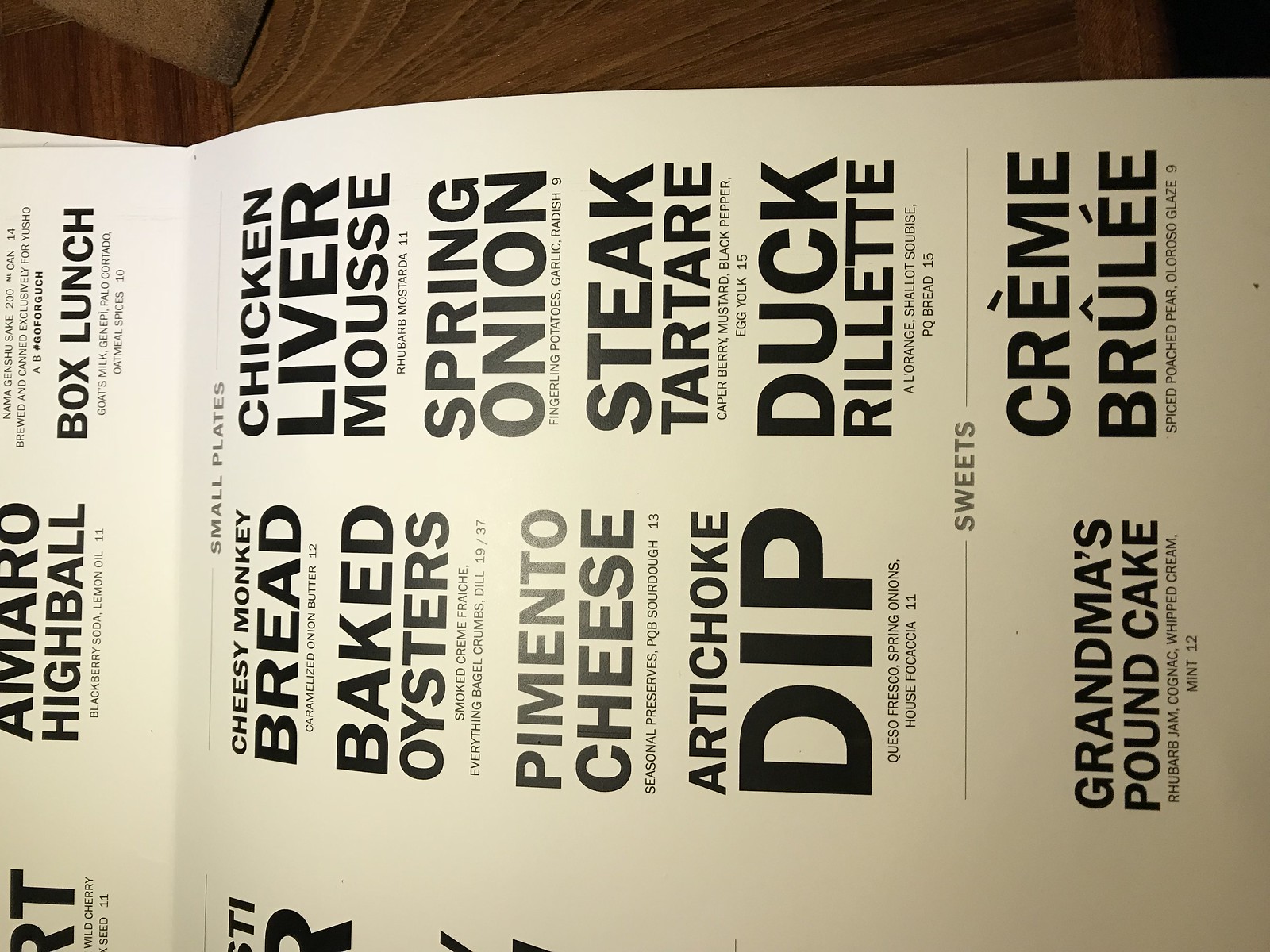The image showcases a menu with an off-white background and black lettering, positioned inside a wooden box with visible horizontal and vertical wood grain patterns. The menu, titled "Box Lunch," is categorized into sections such as "Small Plates" and "Sweets."

The "Small Plates" section includes:
- Cheese Monkey Bread
- Baked Oysters
- Pimento Cheese Artichoke Dip
- Chicken Liver Mousse
- Spring Onion Steak Tartare
- Duck Rillettes

Within the "Sweets" section, the menu lists:
- Grandma's Pound Cake
- Crème Brûlée

On the right-hand side, there is a mention of drinks, specifically "Amaral Highball." The image is slightly tilted, making the left-hand side of the menu difficult to read, suggesting that there may be additional items not fully visible in the photograph. The menu rests against the wooden background, giving it a rustic and cozy appearance.